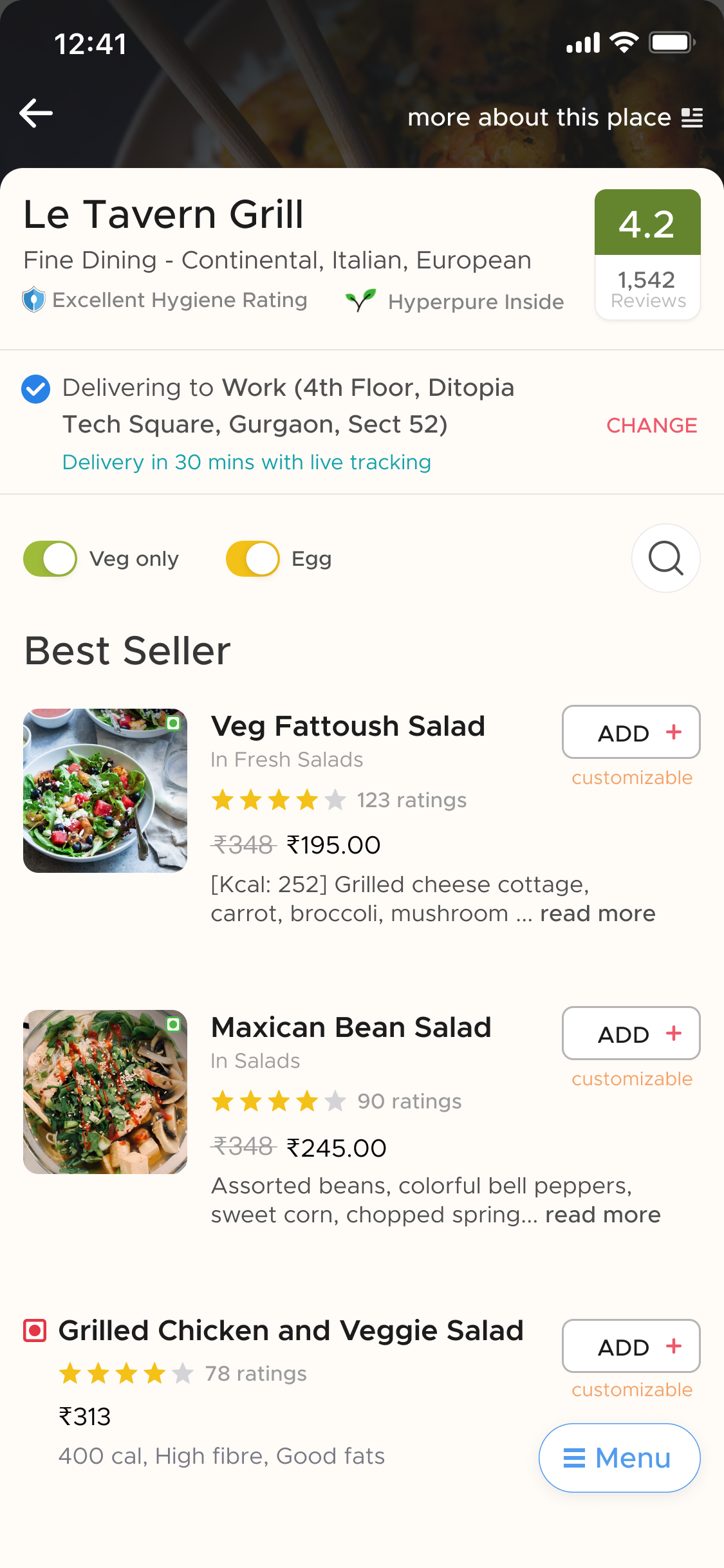Screenshot Details:

**Timestamp and Icons:**
- Time: 12:41 
- Indicators: Mobile network signal, battery status, and Wi-Fi signal on the top right.

**Header Information:**
- **Navigation:** Back arrow on the left side.
- **Section Title:** "More about this place" displayed underneath the status bar.

**Restaurant Information:**
- **Name:** Le Tavern Grill 
- **Cuisine:** Fine Dining, Continental, Italian, European
- **Rating:** 4.2 stars based on 1,542 reviews
- **Attributes:** Excellent hygiene rating, hyper-pure environment

**Delivery Information:**
- **Delivery Address:** 4th floor, Dystopia Tech Square, Gurgaon Section 52
- **Delivery Time:** 30 minutes with live tracking
- **Customization Options:** Vegetarian only or includes egg

**Popular Items:**
1. **Veg Fattoush Salad**
   - **Price:** $195
   - **Calories:** 348
   - **Ingredients:** Grilled Cottage Cheese, Carrot, Broccoli, Mushroom
   - **Availability:** Detailed info available under "Read More"

2. **Mexican Bean Salad**
   - **Category:** Salads
   - **Price:** $245
   - **Ingredients:** Assorted Beans, Colorful Bell Peppers, Sweet Corn, Chopped Sprig

3. **Grilled Chicken and Veggie Salad**
   - **Price:** $313
   - **Calories:** 400